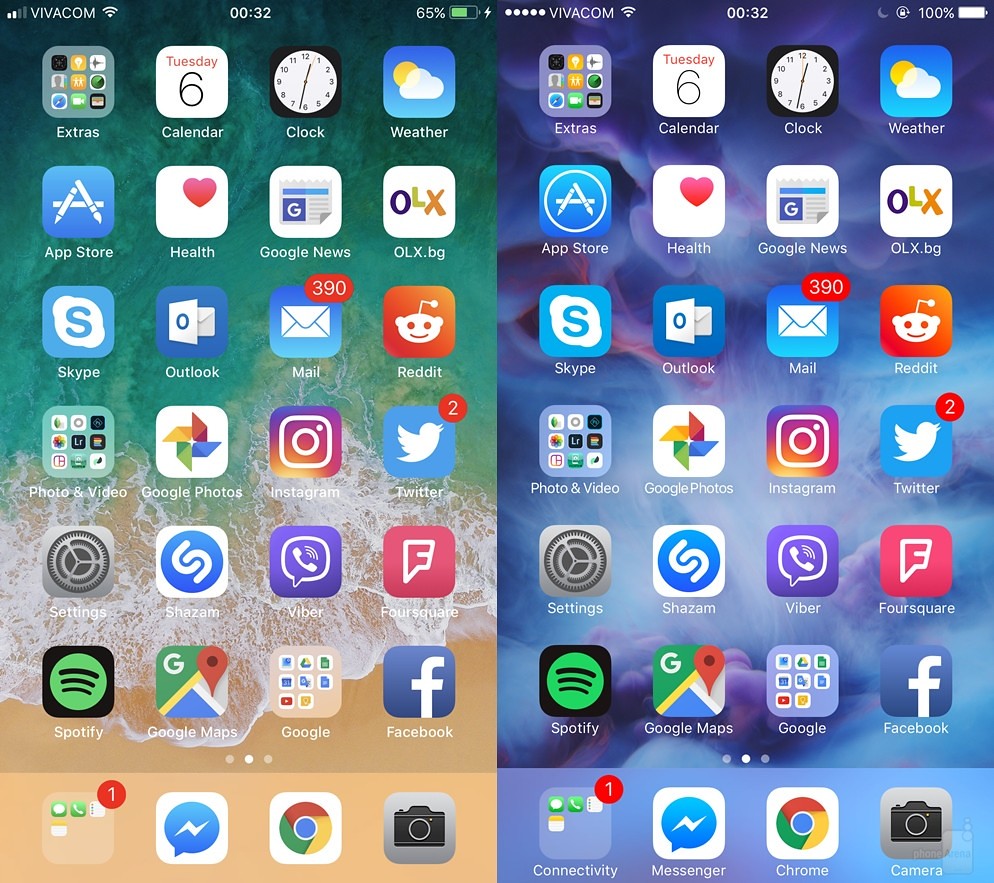A pair of stitched images showcases two nearly identical phone home screens with minor differences. Both screens display "Vivacom" and a white Wi-Fi symbol in the upper left corner. The left screen shows two white bars and two gray bars for signal strength, while the right has five white dots. Centered at the top, both screens feature "0032" in white text. In the top right, the left screen indicates 65% battery with a green icon and a white lightning bolt, whereas the right screen shows a grey crescent moon, a white lock with a circular arrow, a 100% battery with a white icon.

Both home screens contain the same app icons arranged from top left to bottom right: Extras, Calendar, Clock, Weather, App Store, Health, Google News, OLX.bg, Skype, Outlook, and Mail (with 390 notifications). Next are Reddit, Photo and Video, Google Photos, Instagram, Twitter (with 2 notifications), Settings, Shazam, Viber, Foursquare, Spotify, Google Maps, Google, and Facebook. At the bottom, three dots indicate pages, with the middle one white and the others grey. A dock at the screen's bottom features icons for an unlabeled app (with one notification), a blue speech bubble with a white lightning bolt, Google Chrome, and Camera. The right screen labels these icons as Connectivity, Messenger, Chrome, and Camera.

The backgrounds differ: the left screen displays an aerial beach view with yellowish sand, white surf, and light blue water, while the right screen features an abstract cloud-like design in purple and blue hues.